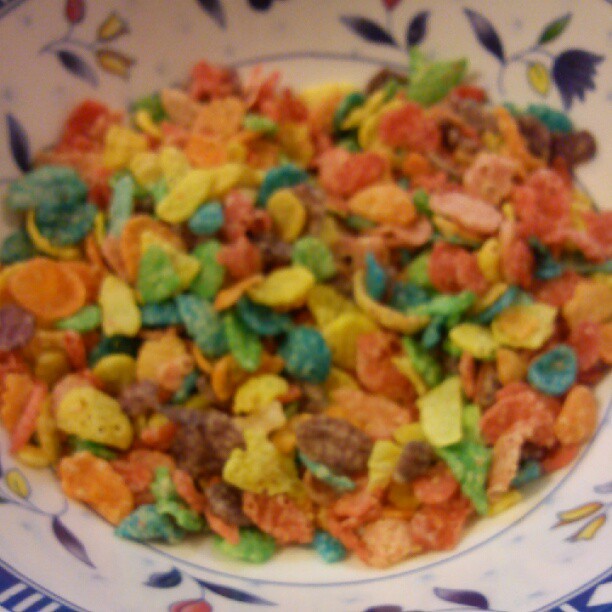This blurry, close-up photograph features a quarter-filled bowl with colorful, multicolored cereal resembling Fruity Pebbles, with pieces in yellow, orange, pink, green, blue, red, and brown. The bowl itself is beautifully decorated with floral designs in blue, yellow, red, pink, and violet, and includes dark blue lines on the inside. Despite the out-of-focus nature of the image, the intricate flower patterns and vibrant hues of the cereal stand out. Notably, the bowl appears to be void of any milk or a spoon.